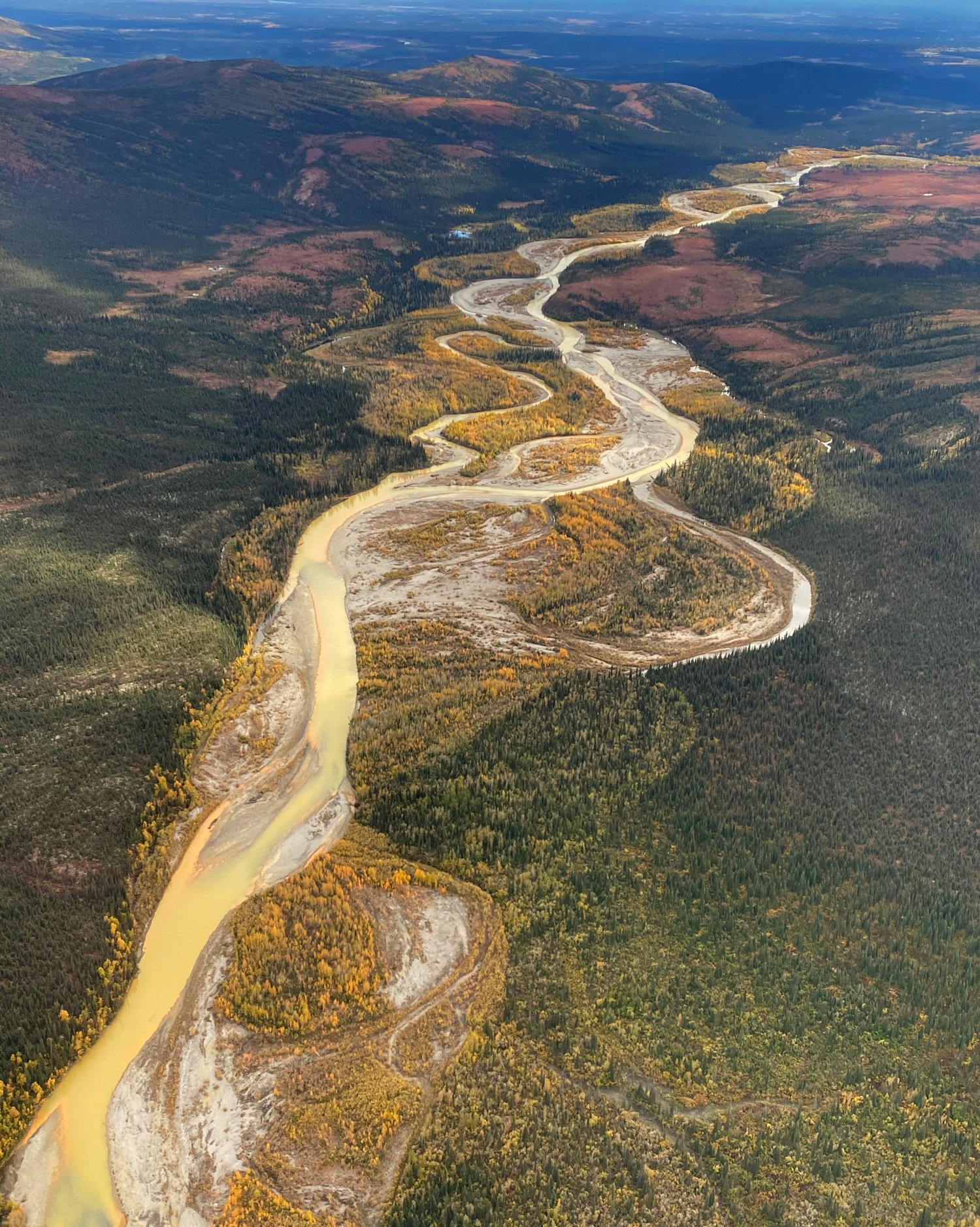This aerial photograph captures a winding river meandering through a valley, bordered by small hills and distant mountains. The river, with its muddy yellow waters, bears evidence of historical shifts in its banks, creating intricate meandering patterns. Surrounding the river, the landscape transitions from verdant green hills to patches of bare earth, indicating recent seasonal changes. The hills showcase a mix of green and brown tones, with the right side abundantly populated by green trees gradually turning golden closer to the river, reflecting the autumn season. Scattered dark green trees accentuate the left side of the valley, enhancing the natural mosaic. Tiny, white rectangular dwellings can be spotted in the distance, adding a subtle human element to the vivid, predominantly natural scene. The overall brightness and clarity suggest it is a clear afternoon, allowing a detailed view of the lush yet varied terrain.